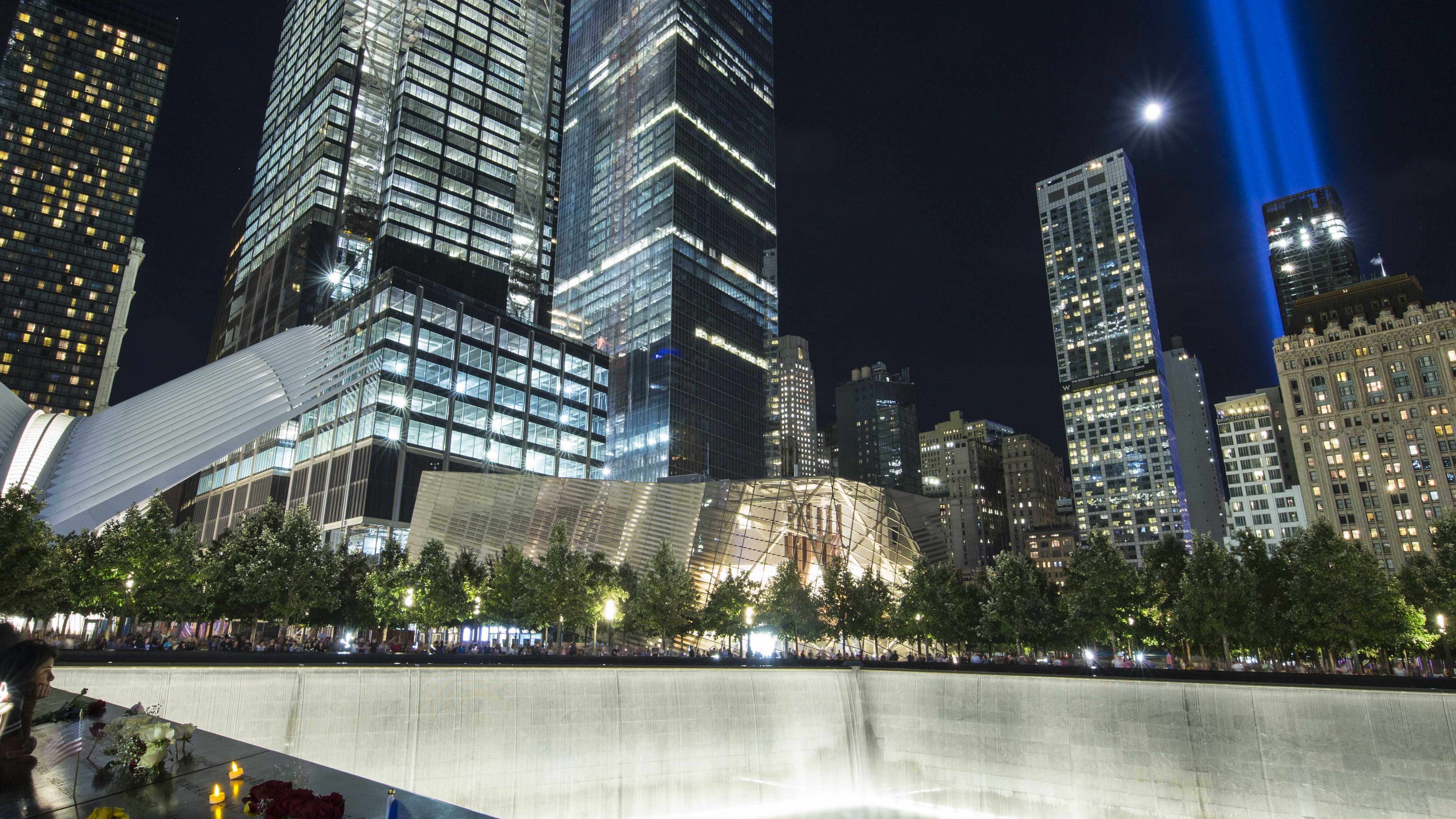This is a detailed nighttime photograph capturing the poignant atmosphere of New York City's World Trade Center Memorial. The image, angled upwards, reveals the illuminated towering buildings that pierce the dark sky. Dominating the top right is a shining full moon, accompanied by two poignant blue beams of light representing the fallen Twin Towers. The foreground features the serene, empty ice skating rink, now marked by the memorial's reflective pools lined with manicured trees that reveal the streetlights below. Surrounding the pools, people gather, their figures silhouetted against the glowing white walls of the footprints of the Twin Towers. Memorial candles and flowers adorn the edges where names are engraved, reflecting a scene likely taken on the anniversary of 9/11. The iconic landmarks of the World Trade Center Museum and the "big bird" building stand prominently in the backdrop, further illuminated by the ambient city lights.